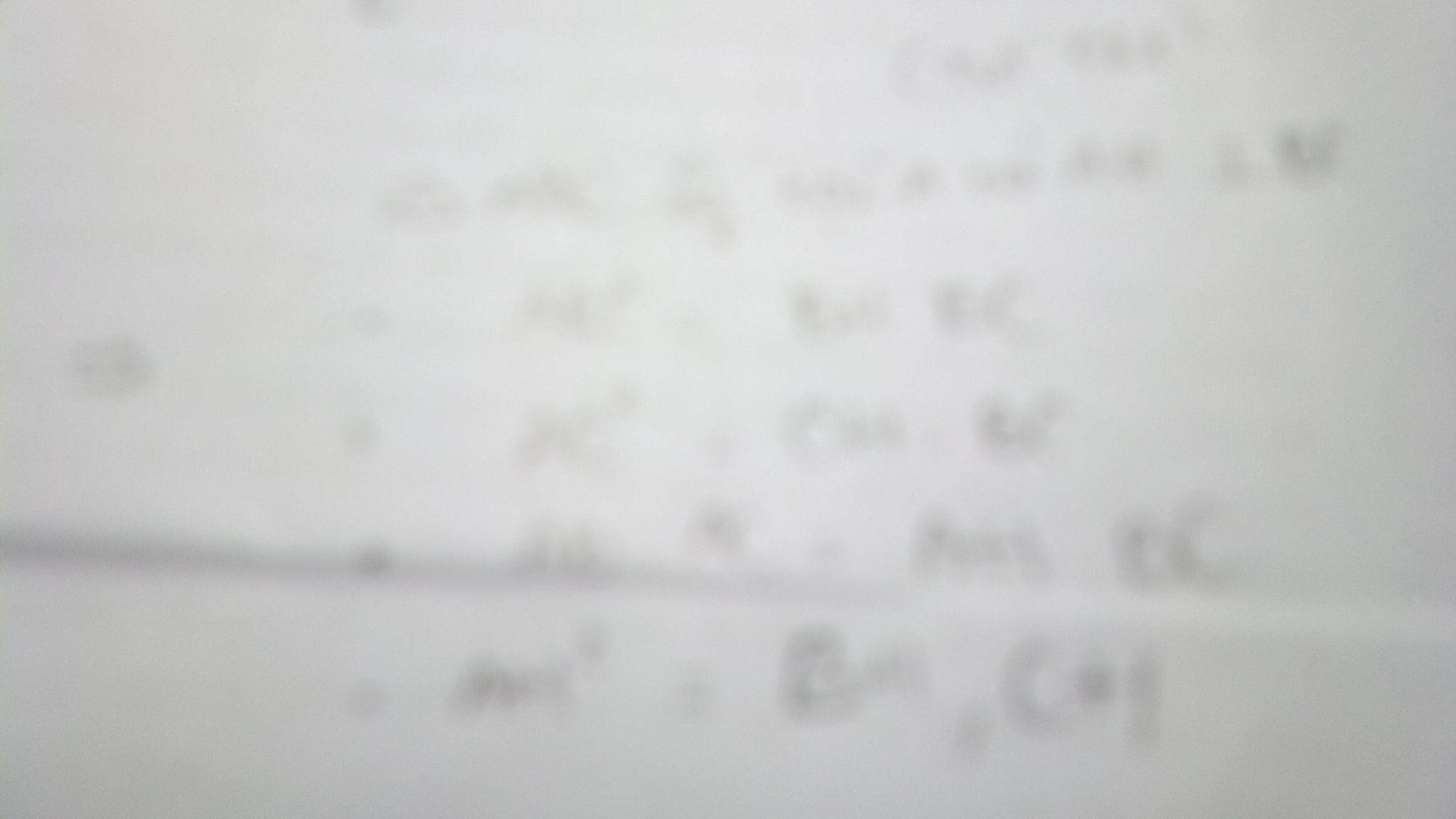This horizontal photograph displays a white sheet of paper with six printed lines of text that are extremely blurred, making the content difficult to decipher. The text appears to be black on the white background. The closest line is vaguely recognizable as potentially containing a mathematical equation, which might include elements such as "m^2 * b...," followed by other unreadable characters. The line above seemingly ends with "cc," while the second line might end with an "m." A prominent, darker, horizontal fold runs across the middle of the paper, indicating it may have been folded. Additionally, on the left side of the paper, there is an indistinct squiggle that could be a mark or another piece of text. Overall, the blurriness of the photo renders the exact details of the text indiscernible.